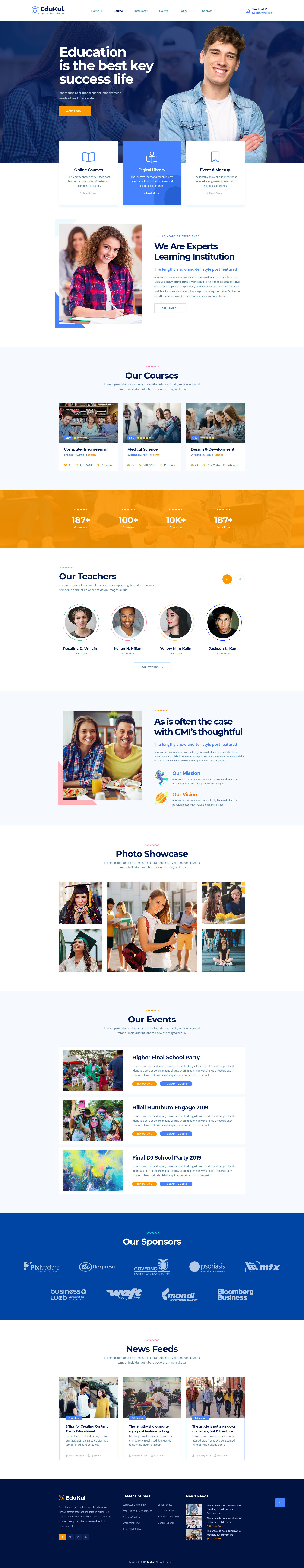The image depicts a webpage that is difficult to interpret due to its low legibility. The header, though mostly unreadable, starts with the word "Education." Below it are two more lines of text that are too blurred to decipher. At the center of the page is an image of a smiling male with short brown hair, wearing a light blue denim shirt over a white tee. The layout consists of three segments in the colors white, blue, and white, each containing some form of text.

Further down, there is a prominent picture of a female, accompanied by a series of smaller images. As you scroll, four smaller individual portraits of different people are displayed. The webpage continues with an assortment of images and various sections, although the specific content remains indistinct. The overall color scheme includes notable accents of blue and orange.